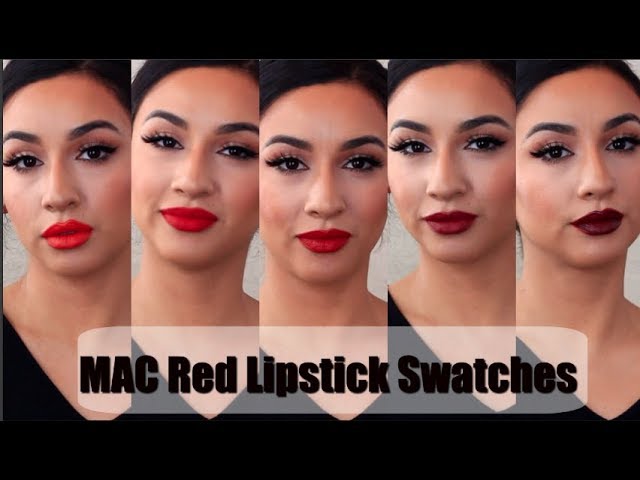The image appears to be an advertisement for MAC Red Lipstick, showcasing five varying shades of lipstick on the same woman. This horizontal rectangular image features a black background with narrow vertical strips, each containing the woman's headshot, lined up from left to right. At the bottom of the image, a transparent white band displays the label "MAC Red Lipstick Swatches" in bold black letters.

The woman sports black hair, tied back with a side part, thick black eyebrows, long black eyelashes, and wears makeup on her eyes. She dons a black V-neck shirt. Each headshot captures her face in slightly different poses, transitioning from a bright red lipstick on the leftmost side to progressively darker reds, culminating in a deep maroon-red on the rightmost side. Her facial expressions vary slightly, ranging from subtle smiles to more neutral looks, enhancing the visual appeal of the lipstick shades.